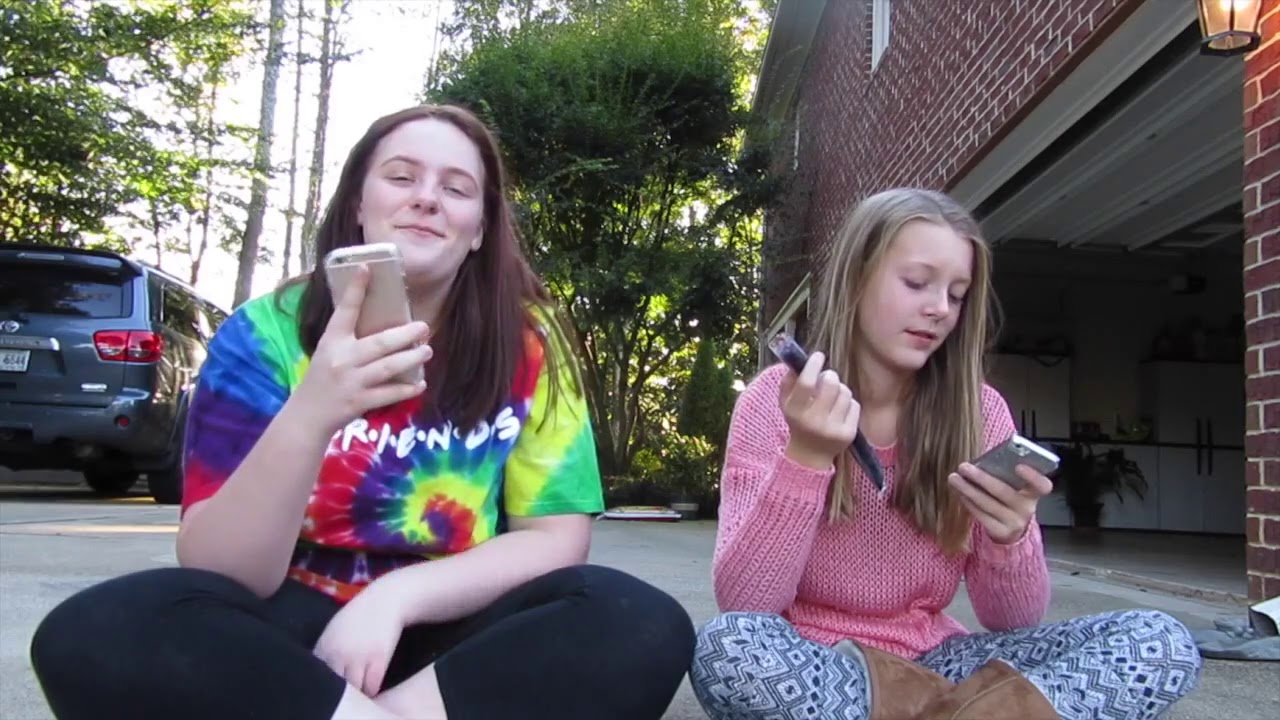In this image, we see a scene set outdoors in the middle of the day, on a paved asphalt driveway in front of a brick, two-story home. Central to the composition are two teenage girls seated cross-legged on the ground, both engrossed in their cell phones. The girl on the left, with straight brown hair cascading to her chest, wears a blue, green, red, and white tie-dyed shirt prominently displaying the title "FRIENDS" from the TV show. She pairs this with black leggings and has a smirk on her face as she looks towards the camera. The girl beside her on the right, with long, straight sandy blonde hair, is dressed in a pink sweater, blue and black tribal print capri leggings, and brown Ugg boots. She is looking down at her phone with a purple ice pop in her hand.

In the background, there is an open garage to the right, indicating the photo was taken in front of a section of the house. This home features a hanging sconce light on the upper right corner of the garage and a white window visible on the second floor. To the left of the girls, we can see the back of a gray SUV, possibly a Toyota, parked facing away from the camera. Trees and a patch of sky can be seen in the distance, adding a touch of nature to the suburban scene. The predominant colors in the image are gray, black, pink, purple, blue, green, yellow, white, and brown.